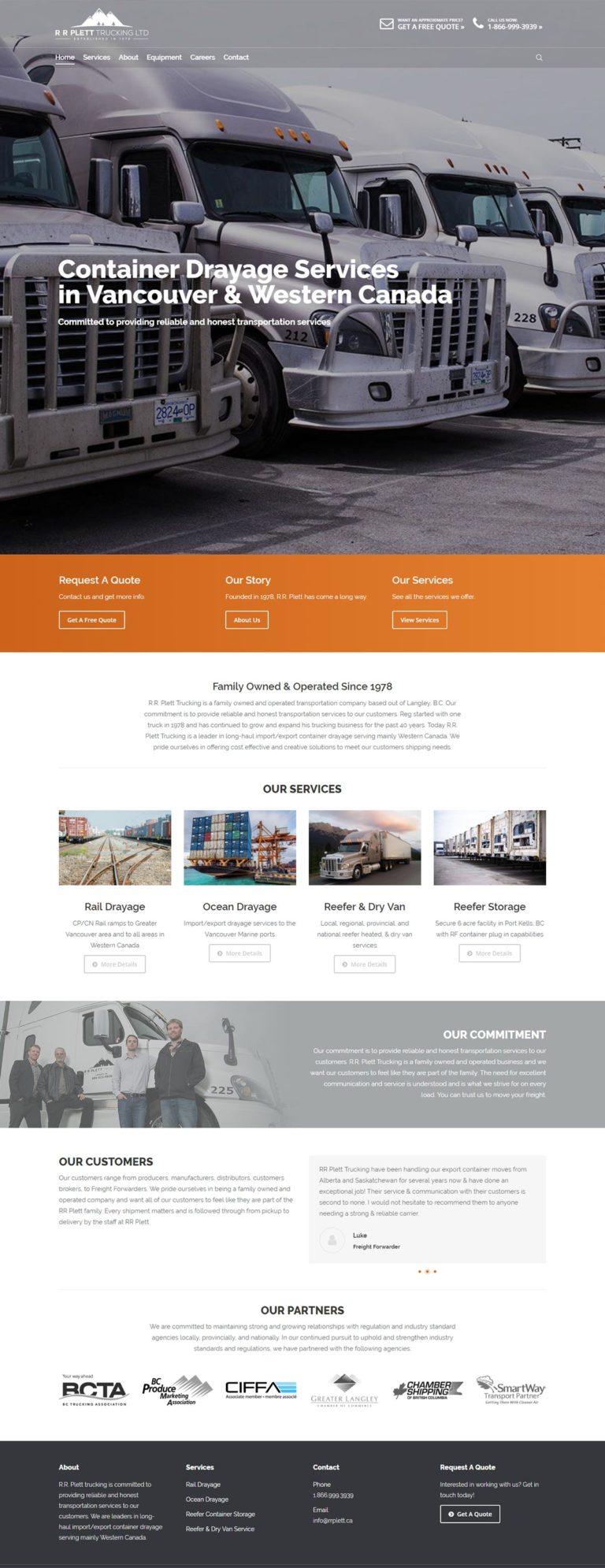The homepage of the RR Platt Trucking LTD website prominently features a large gray banner stretching across the top. In the banner, the company's name, "RR Platt Trucking LTD," is displayed in bold, white letters. Positioned to the right, icons and clickable text provide direct actions: an email icon linked with "Get a Free Quote," a phone icon guiding users with "Call Us Now," followed by the contact number 1-856-999-3939.

On the left-hand side, four imposing 18-wheeler trucks are showcased, revealing only their imposing fronts. Superimposed over these trucks are navigation tabs labeled "Home," "Services," "About," "Equipment," "Careers," and "Contact," all in clean, white letters.

At the center of the trucks, spanning the grilles, is the text "Container Dredge Services in Vancouver and Western Canada." Below this, in smaller letters, is the commitment statement: "Committed to providing reliable and honest transportation services."

At the bottom of the image, an orange "Request a Quote" button stands out, inviting users to get a free quote. This section also features links to other content areas: "Our Story" with a button labeled "About Us," explaining the company’s founding in 1978 and its growth; and "Our Services," with a “View Services” button that leads to detailed descriptions.

Further down the page, smaller images and text describe various specialized services offered, such as "Rail Dredge," "Ocean Dredge," "Reefer and Dry Van," and "Reefer Storage."